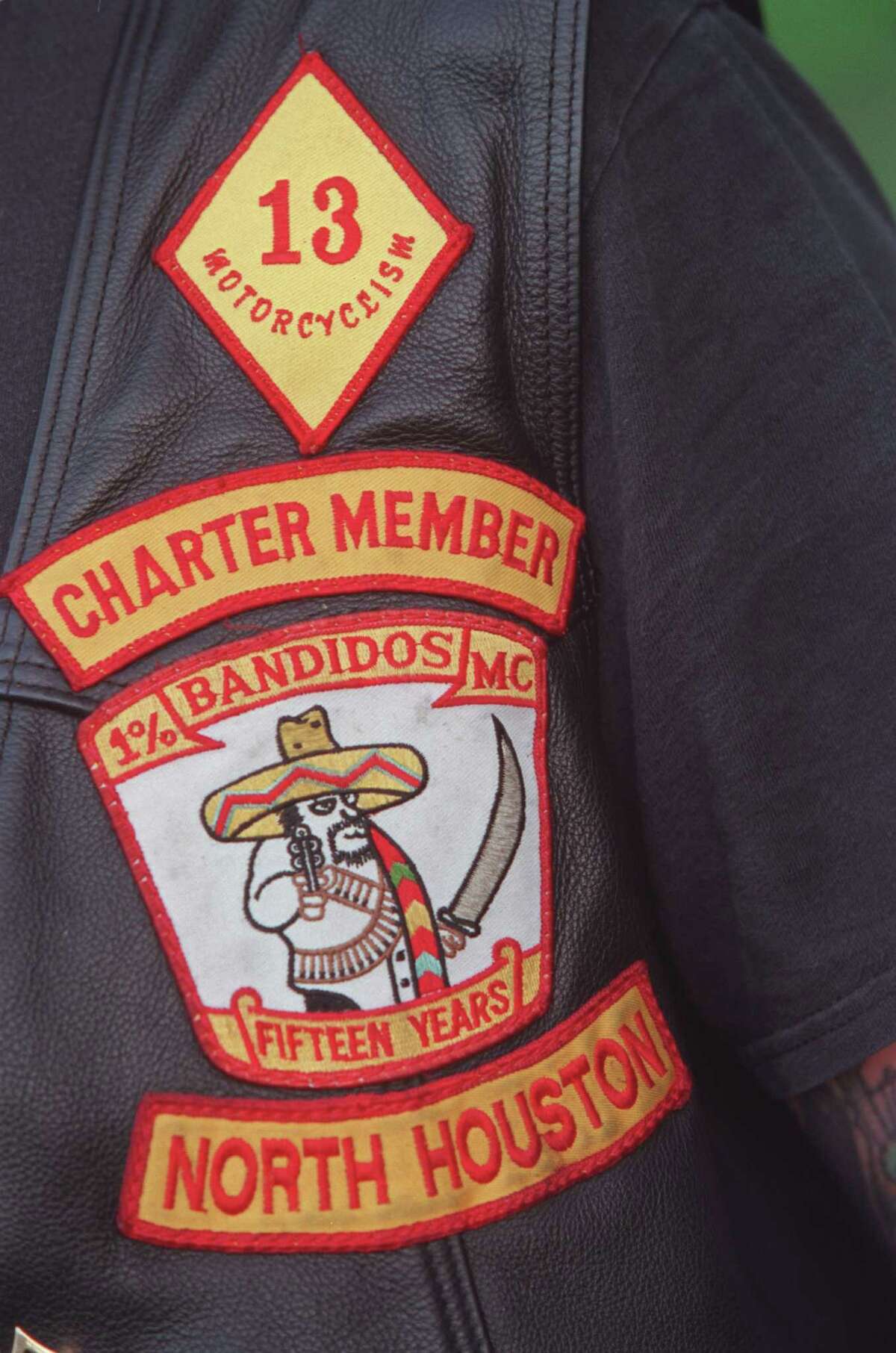The image showcases the patches on a black leather vest worn by a Bandidos Motorcycle Club member. The main focus is the detailed patches emblazoned on the vest. At the top, there's a diamond-shaped patch with "13 Motorcyclism" in red text outlined in yellow. Below it is a ribbon-shaped patch that reads "Charter Member." The centerpiece is a large, intricate patch displaying "1% Bandidos MC Motorcycle Club" alongside "15 years" and features the Bandidos logo—a cartoon figure wearing a sombrero, wielding a sword in one hand and a revolver in the other. Further below is another ribbon-shaped patch that states "North Houston," revealing the member's location. The patches are yellow with red borders and lettering, except for the white background around the logo, which serves to highlight the design further. The member is also clad in a black t-shirt, and a faint glimpse of tattoos can be seen on a small visible part of their arm.